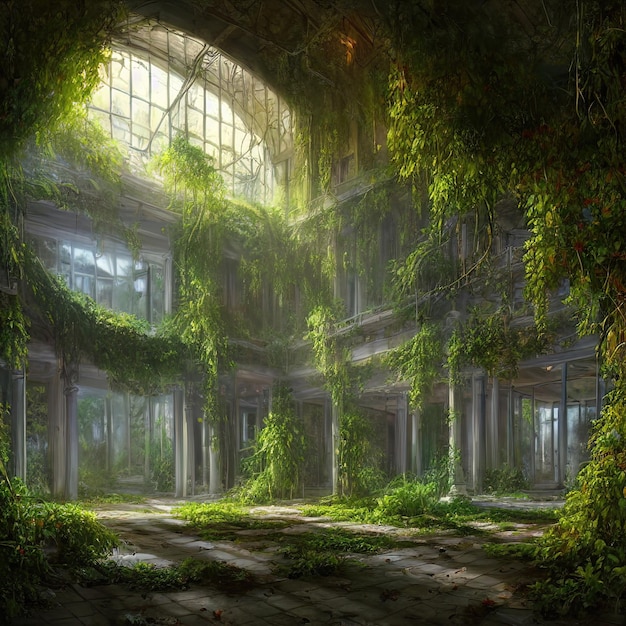The digital illustration, resembling video game concept art, depicts a dramatic and atmospheric scene of an abandoned mall lobby overtaken by nature. The painterly, semi-realistic style showcases a two-story structure with a grand, intact window at the top, allowing sunlight to flood into the space. This light highlights the extensive overgrowth of vines, ivy, and possibly flowering plants that cascade from the ceilings, cling to the tall pillars and posts, and spread across the gray-tiled floor. The vast, empty room, stripped of furniture, exudes a sense of eerie beauty with its enormous glass windows and intricate beams, now draped in greenery. The once grand interior of white walls and beams is almost entirely obscured by the lush vegetation, with occasional glimpses of the original architecture peeking through, suggesting a sense of serenity amidst the ruins.